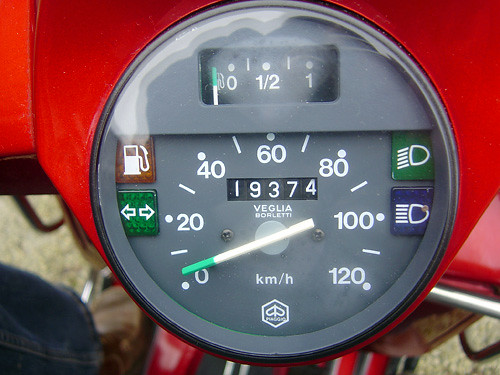This photograph captures a detailed view of a motorcycle speedometer, primarily presented in shades of gray. To the left, a green square with two white arrows pointing in opposite directions signifies the signal indicator. Positioned above it is a red square adorned with a gas pump symbol. The central dial, marked with "KM/H," features white numerals spanning from 0 to 120, with incremental white marks between the numbers.

On the right side of the speedometer, two additional squares are visible: the upper one is green, indicating the headlights facing downward, while the lower one is blue, representing the headlights facing straight ahead. Above these indicators, a rectangular gauge with a miniature gas pump symbol on the left displays fuel levels in white text, marked from 0 to 1, with dashed and vertical lines denoting intermediate levels.

The motorcycle itself boasts a striking candy apple red color and is viewed from an overhead perspective. The underlying ground appears to be concrete, and the image includes the possible knee of the driver on the left-hand side.